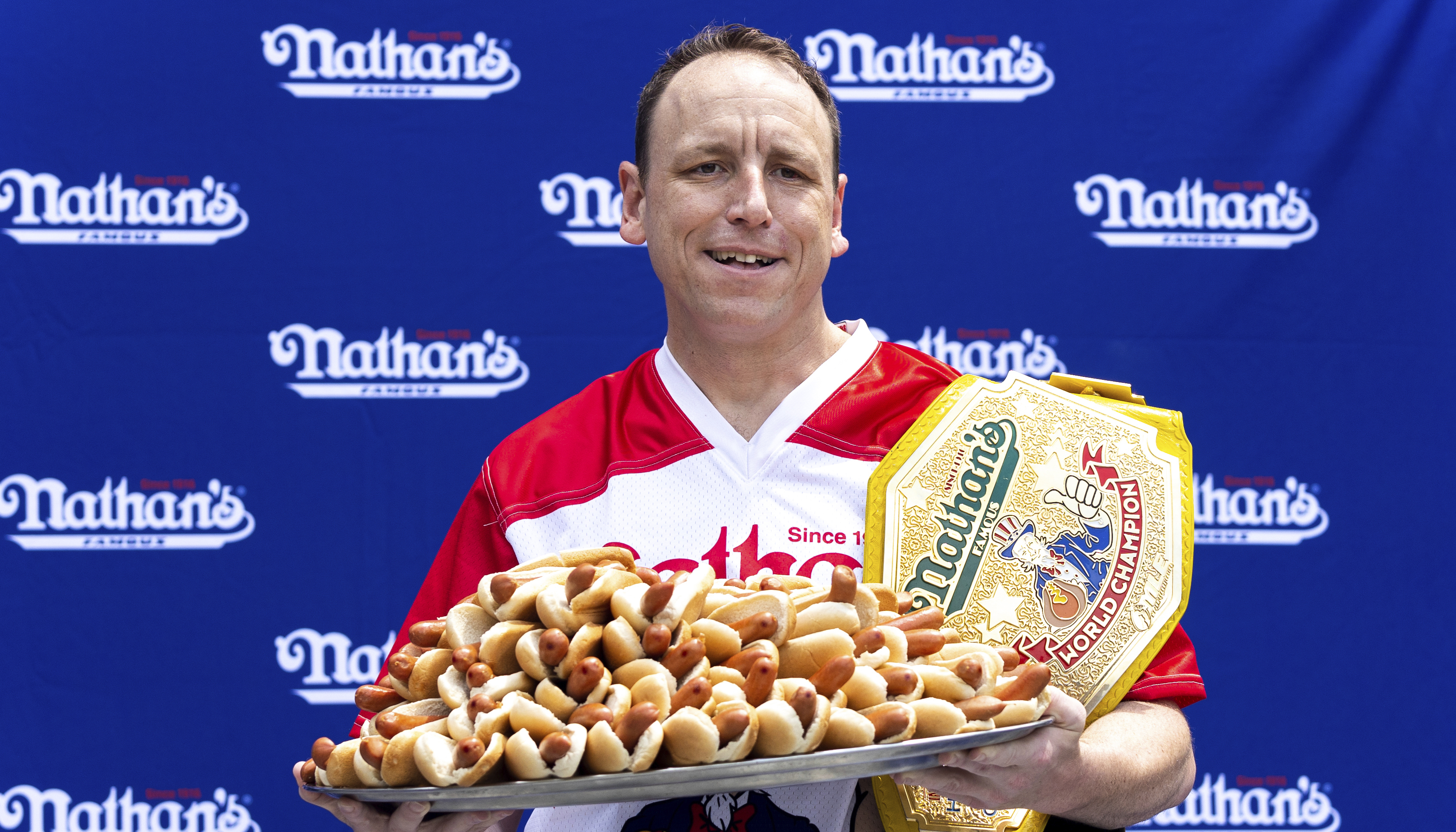In this detailed image, hot dog eating champion Joey Chestnut stands triumphantly at the center, holding a silver platter stacked with approximately 40 hot dogs, each nestled in buns. Joey, a balding man in his 40s, is smiling broadly as he showcases his hard-earned title. He is clad in a white and red jersey that prominently features the Nathan's logo, tying in the iconic imagery of the event. Draped over his left shoulder is the distinguished yellow World Championship belt, emblazoned with "Nathan's Famous World Champion." Behind him, a blue banner repeatedly bearing the white Nathan's logo serves as the backdrop, cementing the setting of the renowned Nathan's Hot Dog Eating Contest held in New York City. The scene captures the jubilant essence of Joey Chestnut's victory in this celebrated competition.